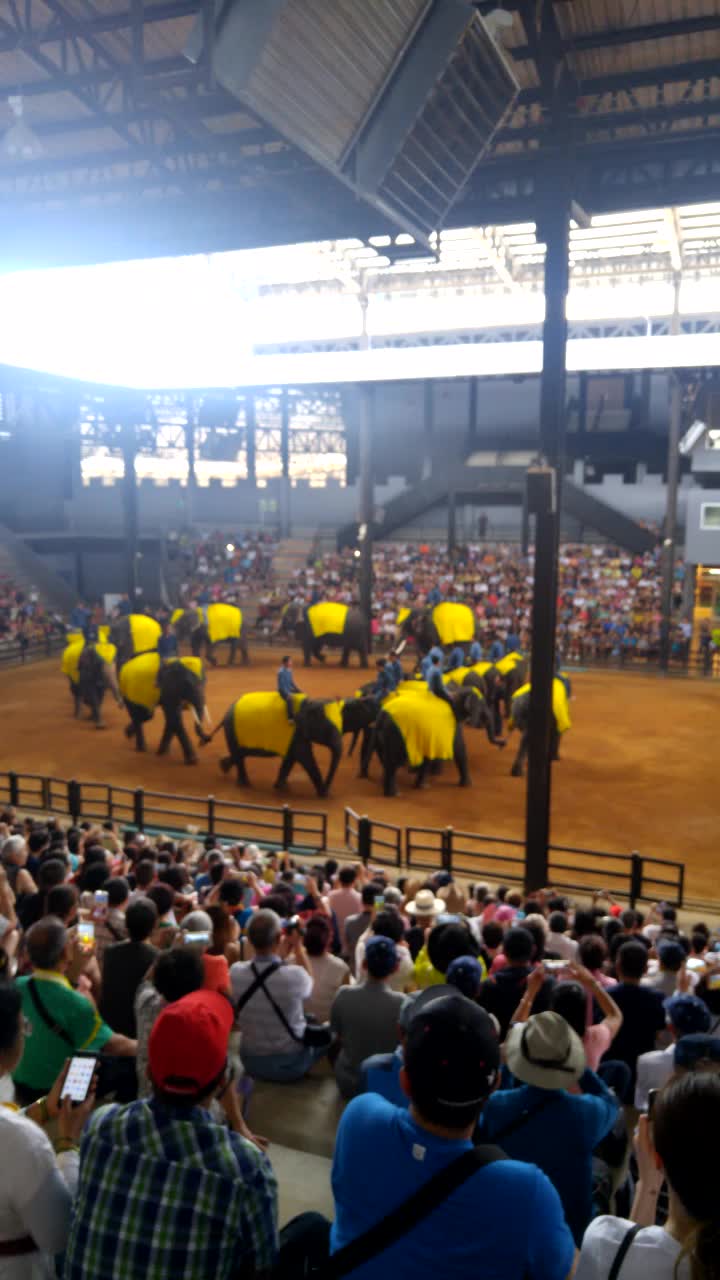The photograph captures a vibrant elephant show from the vantage point of the high-seating area of an open-ceiling arena. The foreground reveals a bustling crowd of onlookers, many adorned with backpacks, likely indicating their status as tourists. The audience is engaged, fixated on the central performance area. The arena's floor is a light burnt sienna brown dirt, surrounded by railings and fencing to ensure spectators are kept at a safe distance.

In the heart of the arena, a group of majestic gray elephants, adorned with yellow blankets draped over their backs, moves in a synchronized circular pattern. Each elephant rider, positioned near the front of the animal close to its neck, is dressed in black pants and a blue long-sleeve shirt. The elephants' long white tusks and graceful trunks add an air of grandeur to the performance. The backdrop of the scene is filled with more spectators on the opposite side of the arena, all intently watching the elephants, creating an atmosphere brimming with excitement and wonder.